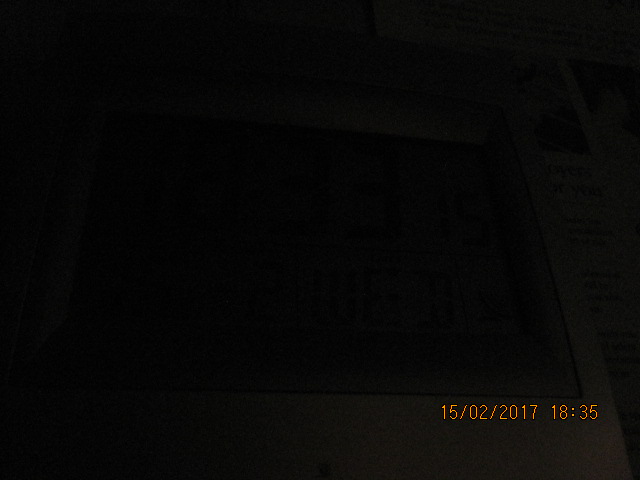This image is predominantly dark and very difficult to discern, with an illumination level of possibly only 5%. At the center of the photo, there is a rectangular-shaped object with a white or light gray border around it, which appears to house a digital clock or timer. The clock's display shows the numbers "3315" or "1033," although it is not entirely clear. This digital clock seems to be positioned on top of a newspaper or magazine, as there is visible text and a black-and-white photograph in the background. The most legible part of the image is a time stamp located in the bottom right corner, written in red or orange text. It reads "15/02/2017 1835," indicating that the photo was taken on February 15th, 2017, at 18:35 (or 6:35 PM in military time).